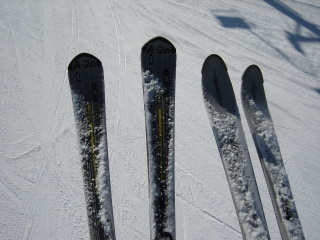This vivid landscape photograph, presented in color, captures a scene typical of looking down from a ski lift ascending or descending a mountain. Prominently positioned in the foreground are two distinct sets of skis, each partially buried in fresh, white snow. Clearly recently used, the skis are divided by a noticeable gap, indicating they belong to two different skiers. The left pair features black tops adorned with a white pattern and a prominent yellow stripe running down the middle. The right pair contrasts with a black base highlighted by a grayish-blue and white texture. The skis, streaked with snow powder, sit above a perfectly smooth snow surface, flawed only by ski tracks stretching out beneath them – evidence of previous skiers gliding over the terrain. Adding to the authenticity of the alpine experience, the top right corner of the image includes a faint shadow of a ski lift and pole, subtly emphasizing the context of the scene.